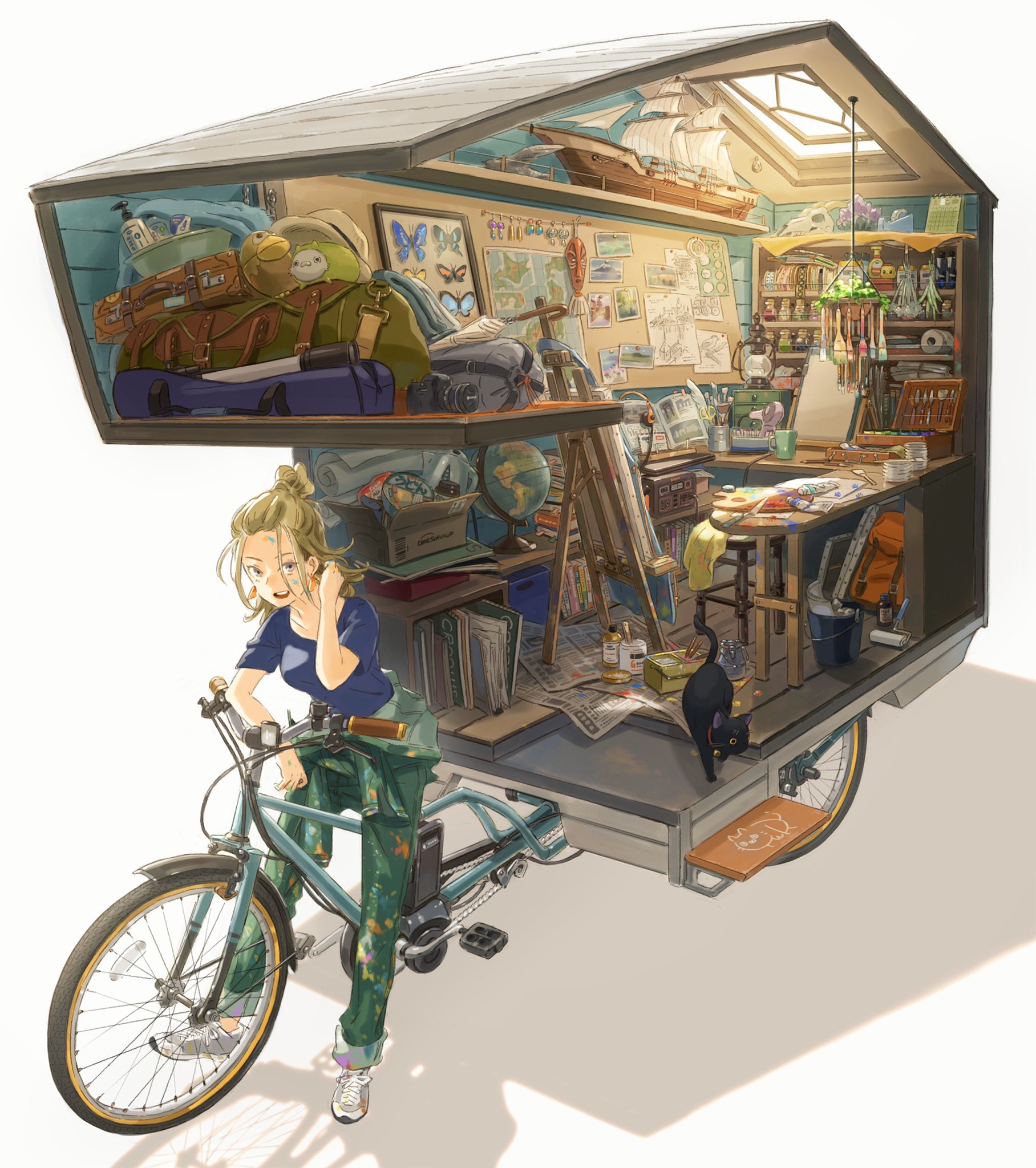In this captivating anime-style illustration, a young girl with her hair tied up rides a custom-built blue bicycle. Attached to the bike is a unique trailer that doubles as her mobile living space. This compact trailer is meticulously organized and serves as her personal sanctuary, complete with a cozy bedroom setup. Inside, a desk sits alongside an easel for her artwork, surrounded by various paints and an array of artistic supplies. A black cat comfortably shares this tiny home on wheels, adding a touch of companionship to her journey. The trailer also features a bulletin board, a backpack, and storage bags, hinting at her nomadic lifestyle. Butterflies flutter around, adding a whimsical touch to the scene. Though there doesn't seem to be an explicit sleeping area, the space is ingeniously utilized to function as both a living quarters and an art studio, reflecting her creative spirit and adventurous life.